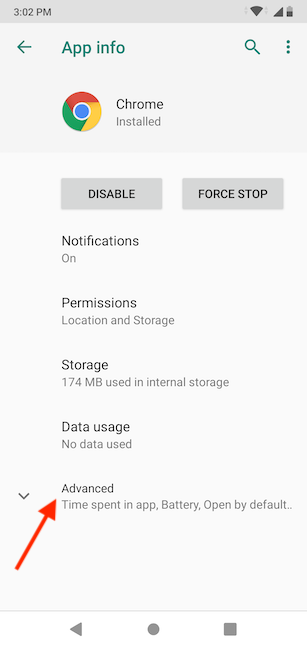A detailed screenshot of the Chrome app information on an Android device. The header at the top is gray, displaying the time at 3:02 p.m. on the left with full Wi-Fi and cell signal indicators, and a battery meter showing approximately 50% charge. To the right, there is a green back arrow, a green 'App Info' label, and a green triple-dot menu. A green (or teal) magnifying glass icon sits next to the Chrome logo and the word "Chrome" followed by “Installed.”

Beneath this header, two side-by-side buttons are visible. The left button says “Disable” in black text on a gray background, while the right button mirrors this design but with “Force Stop” as the label. Further below, there are five options listed, with ample white space between each item. The primary options include "Notifications - On," "Permissions," "Location," and "Storage," with a secondary line underneath the storage indicating "174 MB used in internal storage" in a lighter and smaller gray font compared to the main options.

Following these entries, "Data Usage" shows "No data used," and the final option is "Advanced," which includes sub-options such as "Time spent in app," "Battery," and "Open by default." An overlay in the image features a red arrow angled about 10 degrees to the right, pointing upwards towards the "A" in "Advanced."

At the very bottom of the screenshot, the navigation bar appears with three solid gray icons: a left-facing triangle (Back), a circle (Home), and a solid square (Recent Apps).